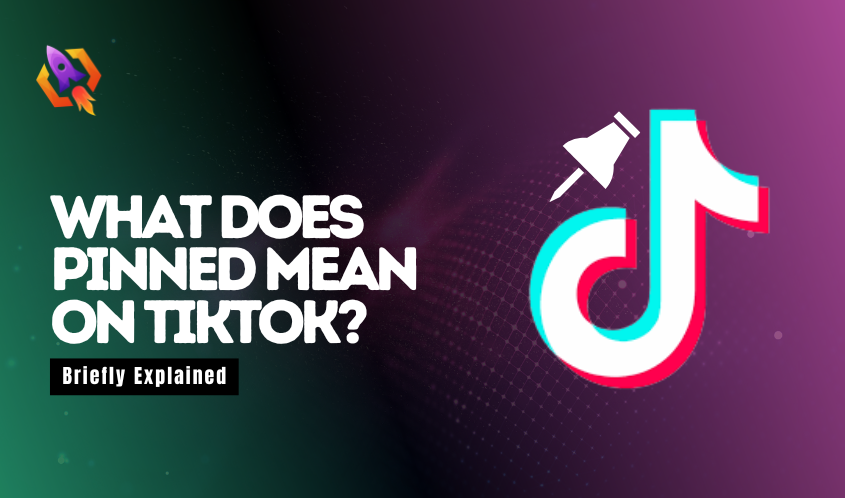This digital artwork features a vibrant, multicolored background that transitions smoothly between different hues. On the left side of the image, a hazy, bluish-green triangle of color begins at the top left and fades into black near the center left at an angle that extends down to the bottom center. This green segment gradually transitions into a purple background on the right side.

The purple section is adorned with a white grid pattern that mimics the curvature of a sphere, with white dots marking the intersections of the grid lines. Scattered across both the green and purple areas, various white dots create the appearance of lens flares, adding a sense of depth and realism to the background.

Prominently displayed in the green area are white, all-caps text arranged in three lines, posing the question: "WHAT DOES PINNED MEAN ON TIKTOK?" Just beneath this text, but slightly to the left, a black rectangle contains smaller white text, also not in all caps, that reads: "briefly explained."

In the top left corner, an orange gradient octagon with a central cut-out showcases a purple rocket icon, complete with orange and yellow flames ejecting from the bottom, symbolizing dynamic motion and energy.

Overlaid on the purple background, near the right, is a logo resembling a musical eighth note. The pink eighth note has a distinctive design where the curl does not completely meet the stem. A blue version of the note is slightly offset above and to the left, creating an overlapping effect that results in a white highlight where the two versions intersect. Just above and to the left of this logo, a white pushpin icon is casually placed.

Overall, the image is not only visually captivating with its vivid colors and dynamic design elements but also informative, posing a question about TikTok functionality while aesthetically engaging the viewer.